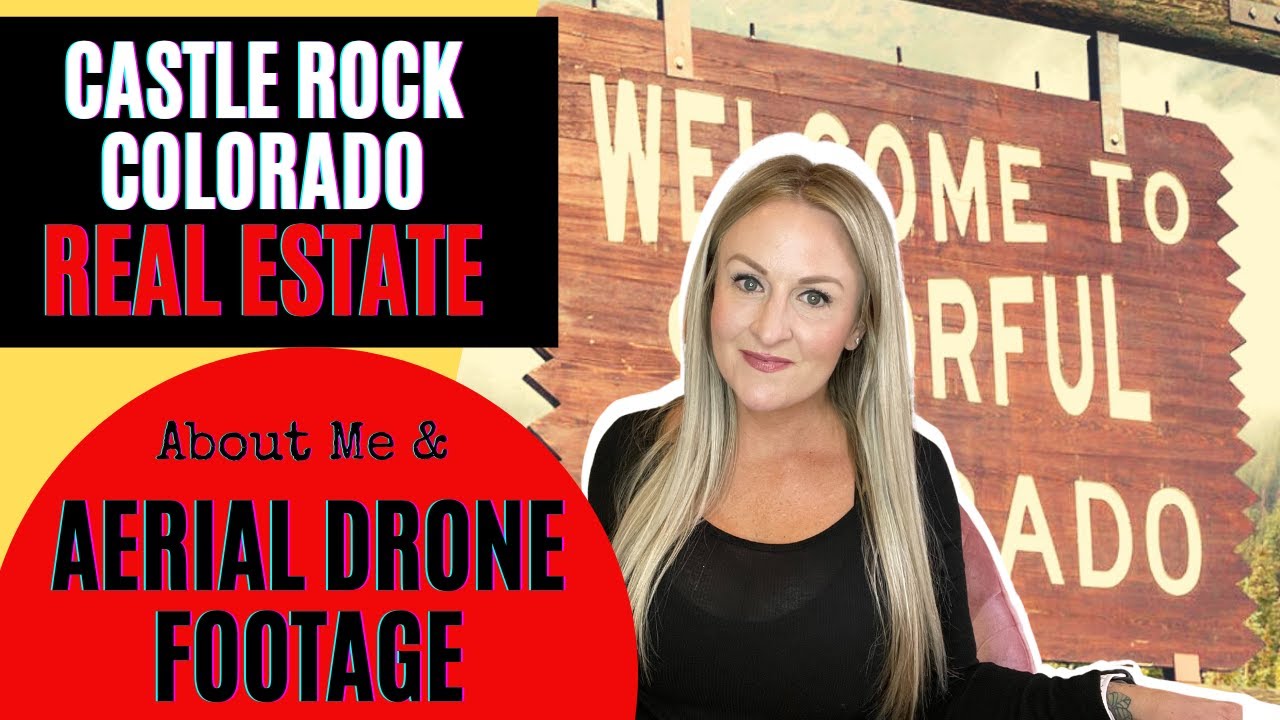In the top left corner of the image, there is a black box with "CASTLE ROCK, COLORADO" written in white, all-caps font, and below it, "REAL ESTATE" in red, all-caps font. Directly beneath this, a red semicircle contains the words "About Me" and "Aerial Drone Footage" in black letters. Adjacent to the semicircle, a photo of a woman with long, straight blonde hair, appearing to be in her early 40s, is shown from the chest up. She is wearing a black blouse and red lipstick, framed by a subtle white outline. Behind her, a partially visible sign reads "Welcome to," followed by the cut-off letters "RF UL" and another line that likely continues the message. This scene suggests she is a real estate agent promoting properties in Castle Rock, Colorado, using both personal branding and aerial drone footage to attract potential buyers.